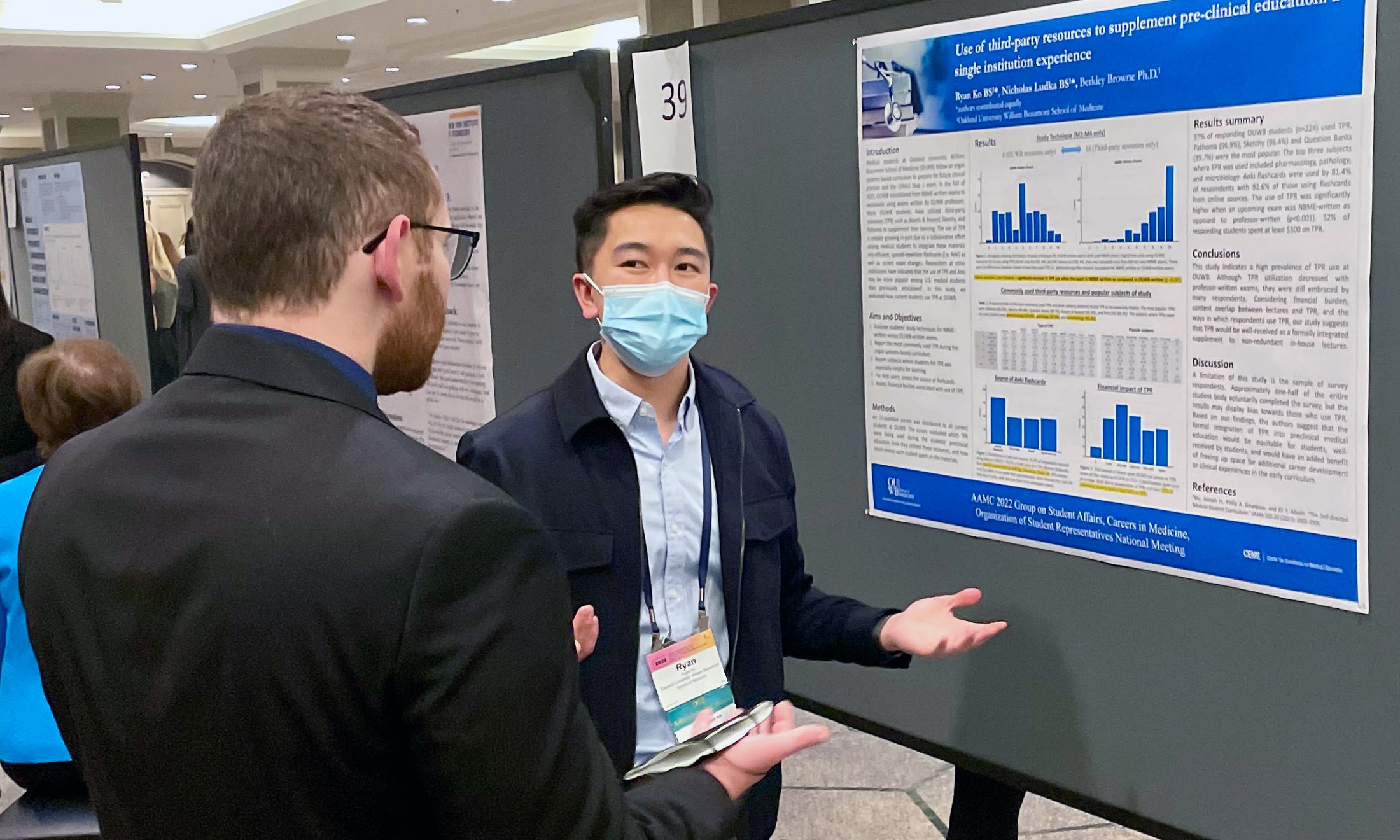The photograph captures a professional setting, likely a trade show or conference, characterized by a large room with visible ceiling elements including possible glass panels and smaller electric lights. In the image, two men are engaged in conversation in front of a grey display board marked with the number 39. 

The man on the left is an Asian gentleman wearing a navy blue suit jacket, light blue button-down shirt, and a surgical mask. He wears a lanyard displaying a professional event tag and has expressive eyes and short, combed hair. He appears to be explaining or presenting information from a poster on the board that features blue bar graphs and various text elements, including "Use of third-party resources to supplement preclinical education in single institution experience."

Standing next to him, on the right, is a white man with his back partially to the camera. He has short brown hair, a reddish beard, and wears black-rimmed glasses along with a black suit. His ear appears noticeably red. Both men are gesturing with open hands as if actively discussing or asking questions about the content on the board.

The board behind them features several blue bar graphs and white and black text, although the fine details are difficult to read. The setting includes additional boards in the background, reinforcing the sense of an organized professional event.